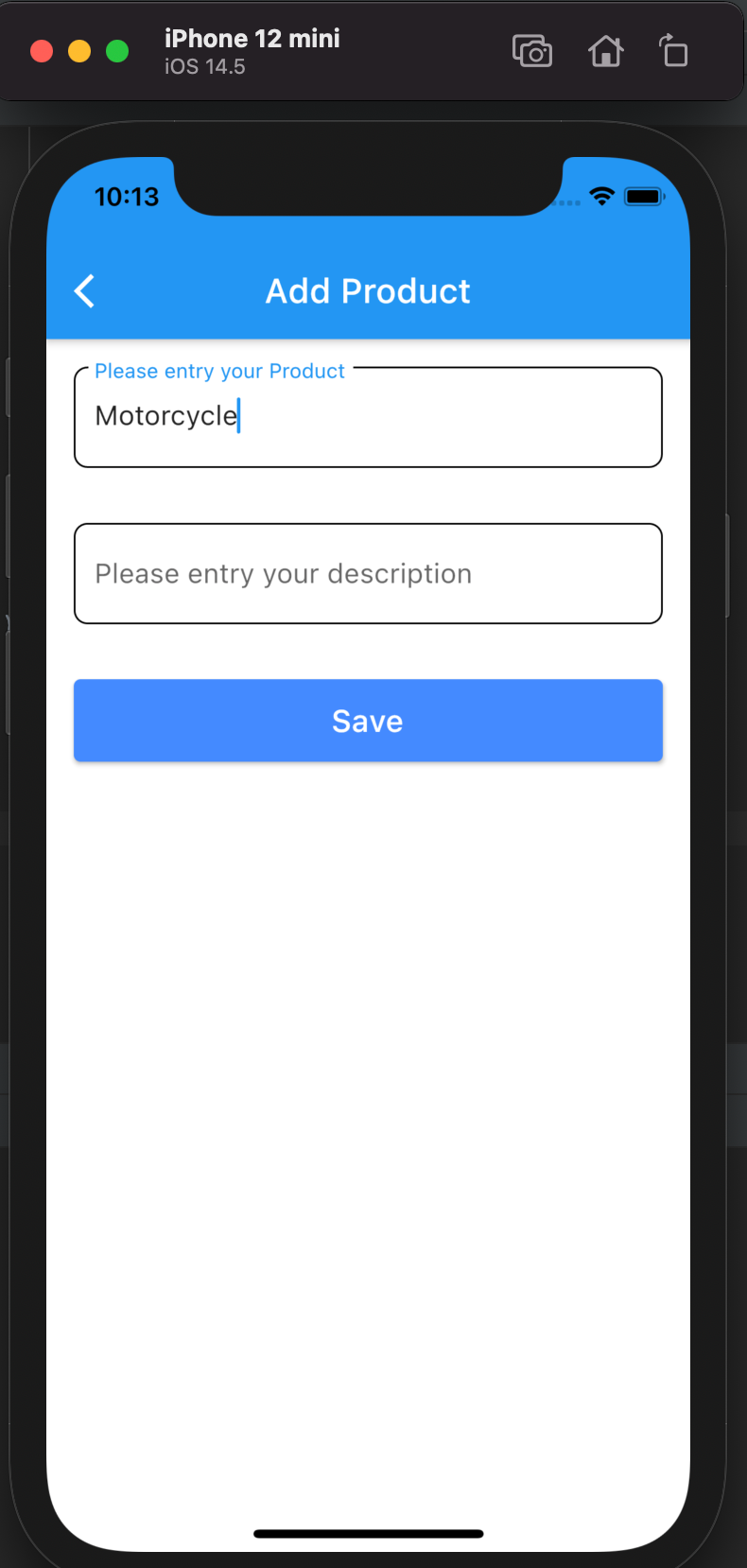### Detailed Caption for Image:

The image depicts a digital interface showcasing an iPhone 12 Mini running iOS 14.5. At the top of the image, "iPhone 12 Mini" is prominently displayed in bold white lettering, with "iOS 14.5" in a lighter gray underneath. To the right, a series of gray icons are visible: a camera icon, a square background, a home icon, and a square with a curved arrow pointing to the right. On the left side of this header, traditional browser control buttons — a red circle, a yellow circle, and a green circle — are visible, indicative of an Apple product.

The central part of the image features an iPhone Mini, recognizable by its standard design and black exterior border. The top of the iPhone screen displays a medium-blue header with the text "Add Product" in white and an arrowhead pointing left. On the very top left of the screen, the time is shown as "10:13" in black, with four signal dots, a black Wi-Fi symbol, and a black battery icon — suggesting the battery is nearly full — toward the right.

Below the header, the iPhone screen has a white background with two editable fields outlined in black with rounded corners. The first field contains blue text that says "Please enter your product," with the word "motorcycle" typed in by the user, and a blue cursor indicating they are still typing. The second field has gray placeholder text reading "Please enter your description." At the bottom of the screen, there is a prominent blue button labeled "Save" in white lettering.